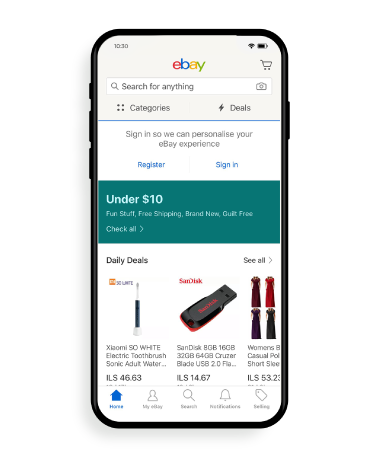This image captures a detailed screenshot of an iPhone displaying the eBay homepage. At the top of the screen, it's 10:30 AM, indicated next to the Wi-Fi symbol and a battery icon showing 75% charge. Below, the familiar eBay logo appears in red, blue, yellow, and green. Icons for a shopping cart, search bar labeled "Search for anything", and various navigation tabs follow.

The page features a variety of sections starting with "Categories" marked by four dots. Adjacent to it, "Deals" is signified by a lightning bolt icon. Further down, a banner invites users to "Sign in" or "Register" to personalize their eBay experience.

Prominently displayed beneath is a banner showcasing items "Under $10" with enticing promises like "Fun stuff, free shipping, brand new, guilt-free". Below this, the "Daily Deals" section highlights featured products: an electric toothbrush priced at $46.63, a SanDisk USB stick for $14.67, indicated with "ILS" (suggesting a currency format), and women's short sleeve dresses for $53.23. Each product is accompanied by a "See All" button to the right.

At the bottom of the screen, essential navigation options are visible: Home, Profile, Search, Notifications, and a final tab, possibly for Tags. The image encapsulates a detailed view of a user's eBay browsing experience on a mobile device.